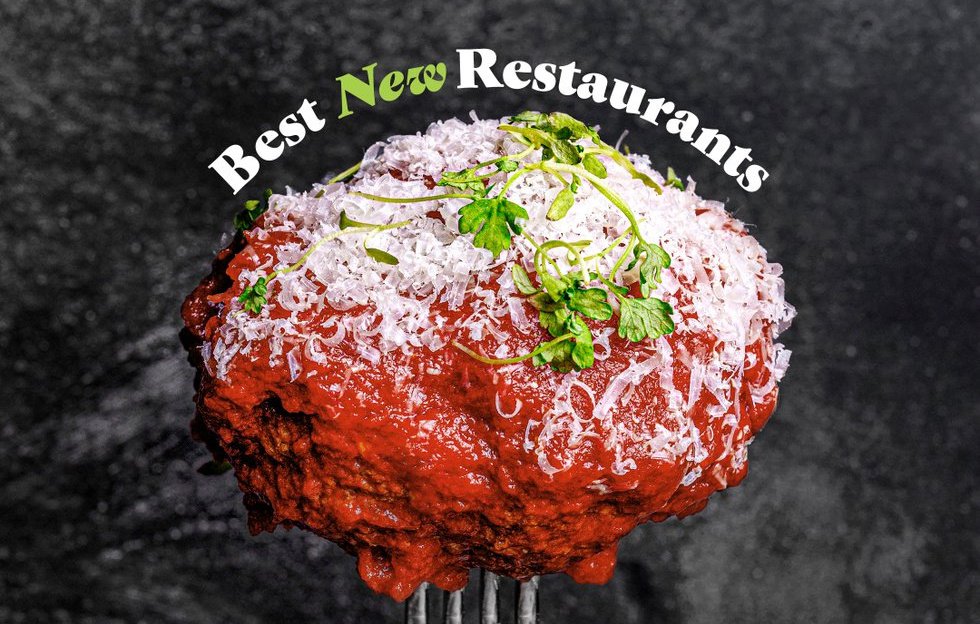The advertisement image is a horizontally aligned rectangular photo featuring a central, prominently displayed meatball drenched in rich tomato sauce and topped with a generous sprinkle of Parmesan cheese and parsley leaves. The meatball, irregular and textured, is held up by a silver fork, the tines of which are visible towards the bottom of the image. Arched above the meatball in bold bubble letters are the words "BEST NEW RESTAURANTS" with "BEST" and "RESTAURANTS" in white, and "NEW" in green. The background is a blurred, granite marble-like texture in varying shades of gray, with darker tones on the left and lighter on the right, adding a sophisticated and moody backdrop to the eye-catching centerpiece.